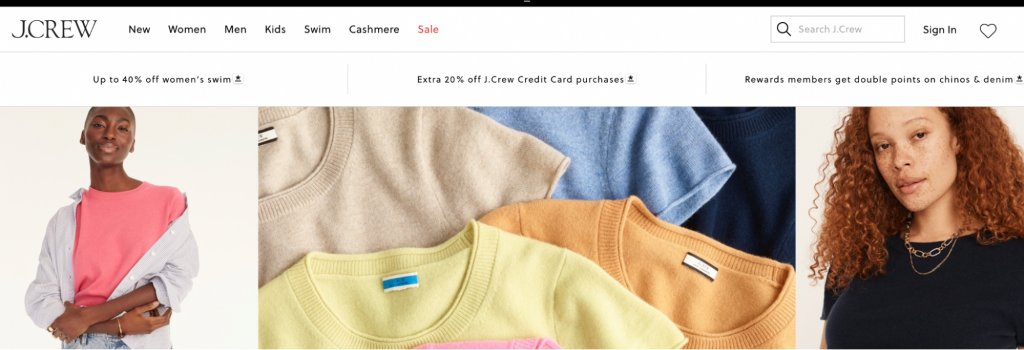A detailed screenshot of the top section of the J.Crew website, featuring a sleek and clean design. In the upper left corner, the recognizable J.Crew logo is prominently displayed. A thin black bar runs across the full width of the top section, providing a subtle yet sleek separation above the main content area, which is characterized by its pristine white background. Adjacent to the J.Crew logo is an accessible navigation menu with categories: New, Women, Men, Kids, Swim, and Cashmere, followed by a striking red "Sale" indicator.

On the right side of the screen, there is a search field accompanied by a magnifying glass icon, inviting users to "Search J.Crew." To the right of the search field, there are sign-in and heart buttons, facilitating user account access and wishlist management. Below the primary navigation area, promotional information is centrally aligned, featuring messages such as "Save up to 40% on Women's Swim," "Save an extra 20% off with J.Crew credit card purchases," and "Rewards Members get double points for chinos and denim."

The visual layout includes two square photos flanking a larger, wider photo in the center. On the left is an image of a black woman with a shaved head, smiling warmly and dressed in a pink top with a light lavender, possibly dress shirt or cardigan, paired with jeans, her arms confidently folded. On the right is a woman, potentially African-American or mixed race, with light skin, freckles, and red hair, donning a tight blue short-sleeved t-shirt and a gold chain necklace. The central image showcases an array of short-sleeved t-shirts, or perhaps fleece shirts with cut-off, rolled-up sleeves, in a palette of beige, light blue, orange, yellow, and dark blue hues, giving a hint of casual and comfortable fashion options available on the site.